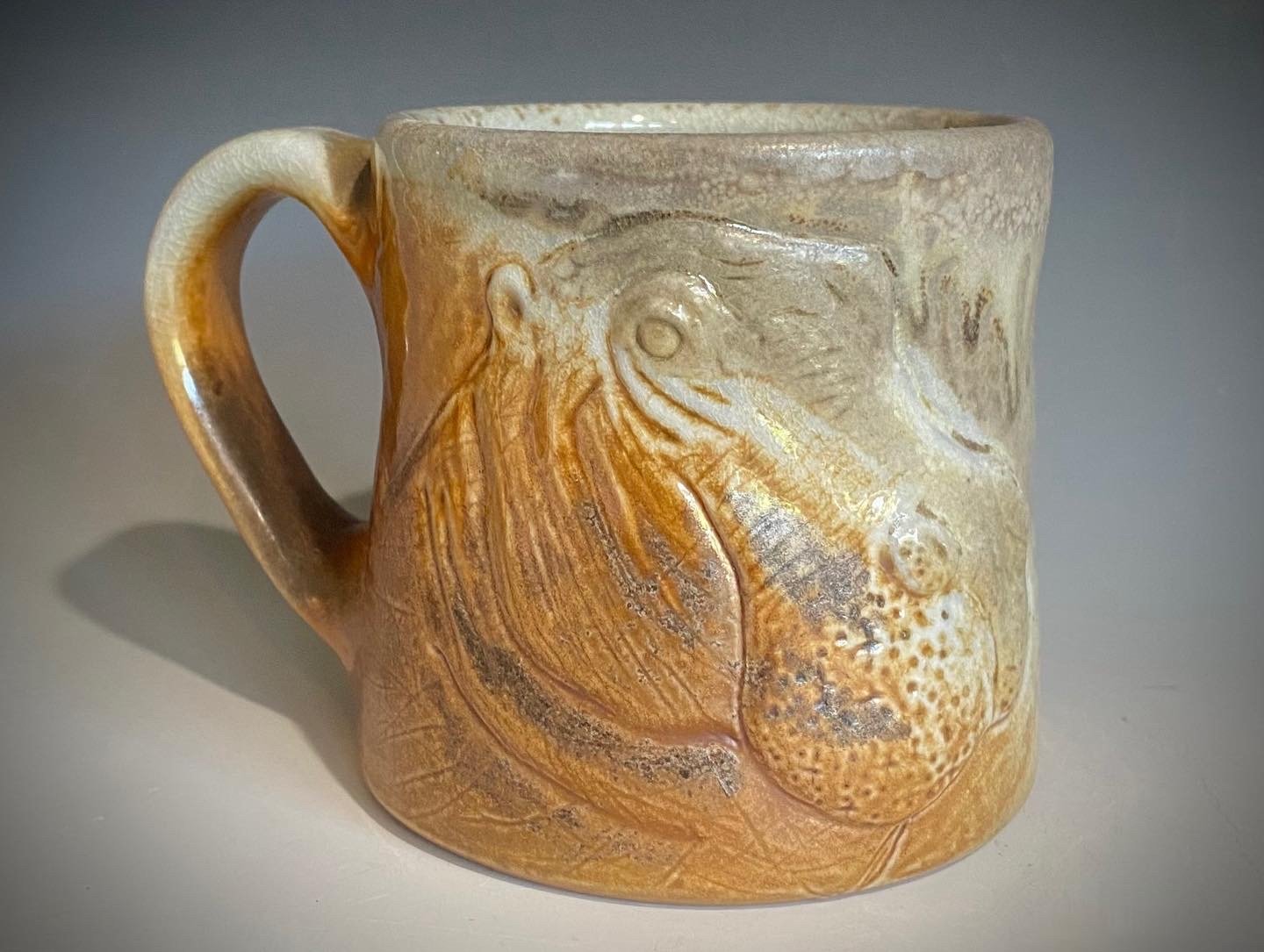This photograph depicts a ceramic mug with an aged appearance, set against a plain gray background. The mug features a diagonal two-tone design, with the lower portion in an orangish-brown hue and the upper part in a whitish-gray shade that extends into the interior, which also appears gray. Prominently displayed on the mug is a detailed relief of a hippopotamus, showing its face slightly turned toward the viewer with a fierce expression. The handle of the mug follows the same color scheme, being mostly brown with a white top. The intricate craftsmanship and unique coloration suggest it might be a vintage or artisanal piece.